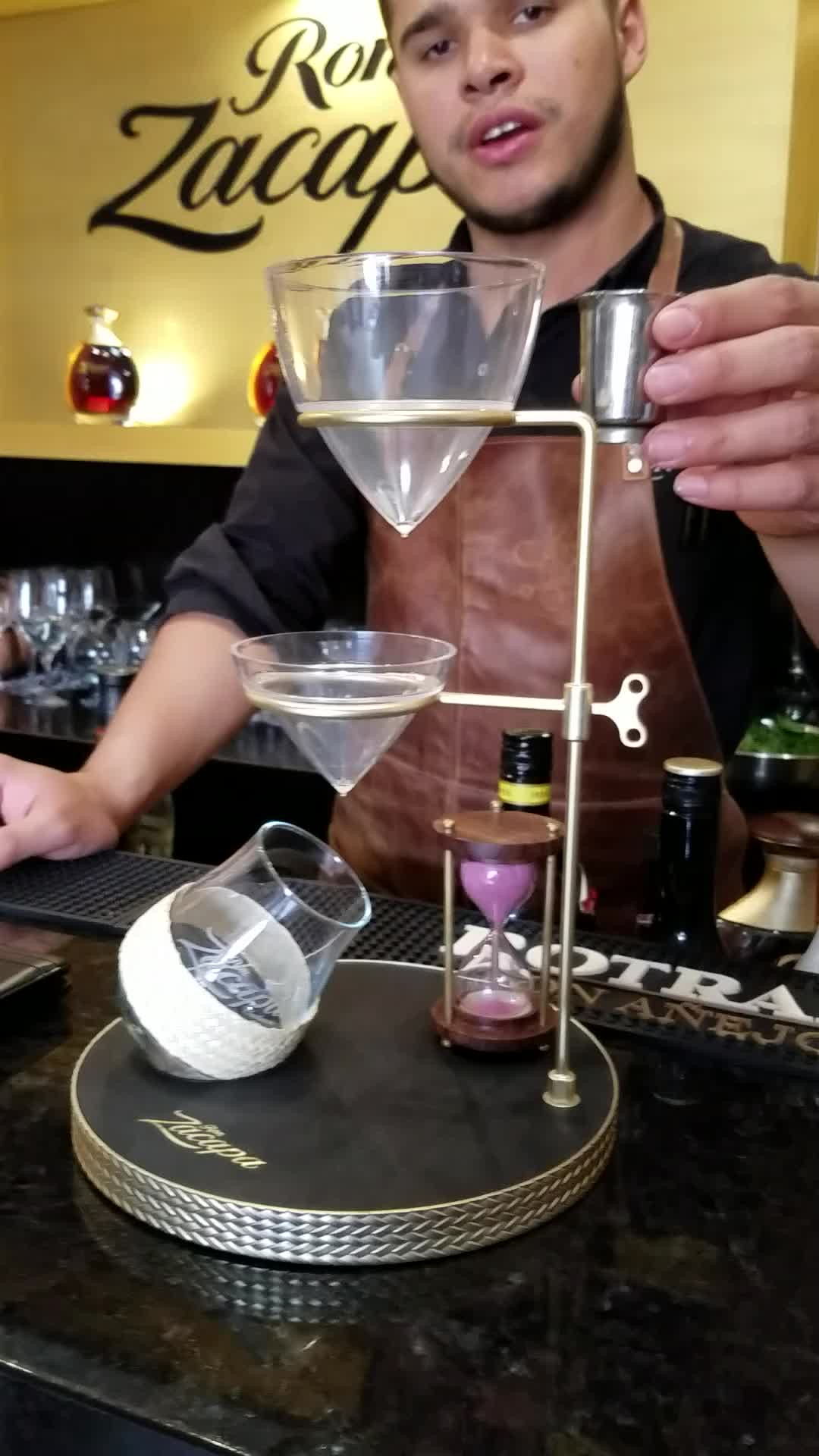The image depicts a man standing behind a dark stone service counter in what appears to be either a restaurant or a coffee shop. He has a medium-light complexion, dark eyes, a patchy thin mustache, and very short hair, and seems to have not shaved for a couple of days, giving him a slightly rugged appearance. Dressed in a black polo shirt and a brown, leather-like apron, possibly as part of his uniform, he holds a small metal tumbler in his right hand. 

In front of him on the counter is a notable contraption that features a metal base with a round platform. Attached to the platform are poles that hold two triangular-shaped glass containers arranged like funnels, intended for some sort of filtering process. Also on the base is a small hourglass timer filled with lavender-colored sand, likely used to time short intervals. 

Behind the man, the background features a gold wall adorned with various bottles and stemware, with the visible partial lettering "ROZACAP" suggestive of a branding or signage. The overall setting suggests a stylish, modern atmosphere typical of a sophisticated beverage establishment.